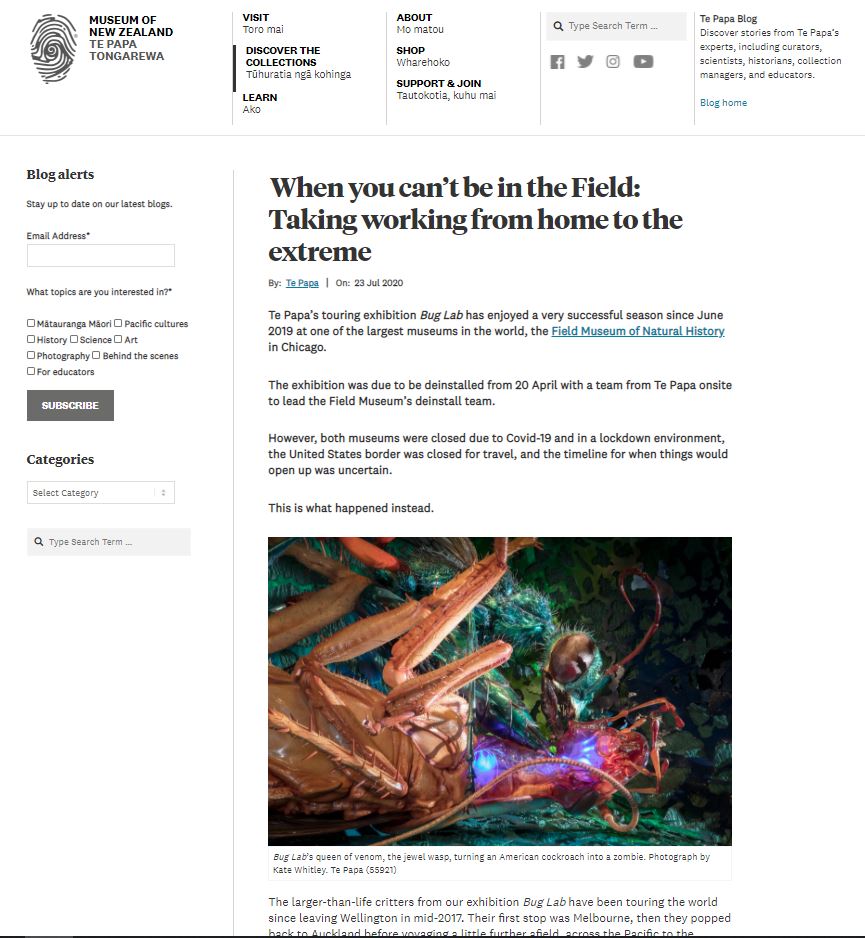**Descriptive Caption:**

Explore the Museum of New Zealand Te Papa Tongarewa from the comfort of your home. Our virtual experience offers you the chance to visit Toro Mall, discover our extensive collection, learn about diverse exhibits, shop for unique items, support the museum, and join our community. Utilize our search box for easy navigation and stay connected through our social media platforms on Facebook, Twitter, Instagram, and YouTube.

Amidst the global pandemic, traditional fieldwork and museum visits have shifted dramatically. Reflecting this change, our "Te Papa Tour and Exhibition" featuring the highly acclaimed Bug Lab has enjoyed a successful run since June 2019 at the Field Museum of Natural History in Chicago, one of the largest museums in the world. Originally scheduled for de-installation on April 20th, the process was halted due to COVID-19-related closures and lockdowns. With both museums shutting their doors and international travel restrictions in place, the timeline for resuming normal operations remains uncertain. Despite these challenges, we continue to innovate and bring extraordinary experiences to you, wherever you are.